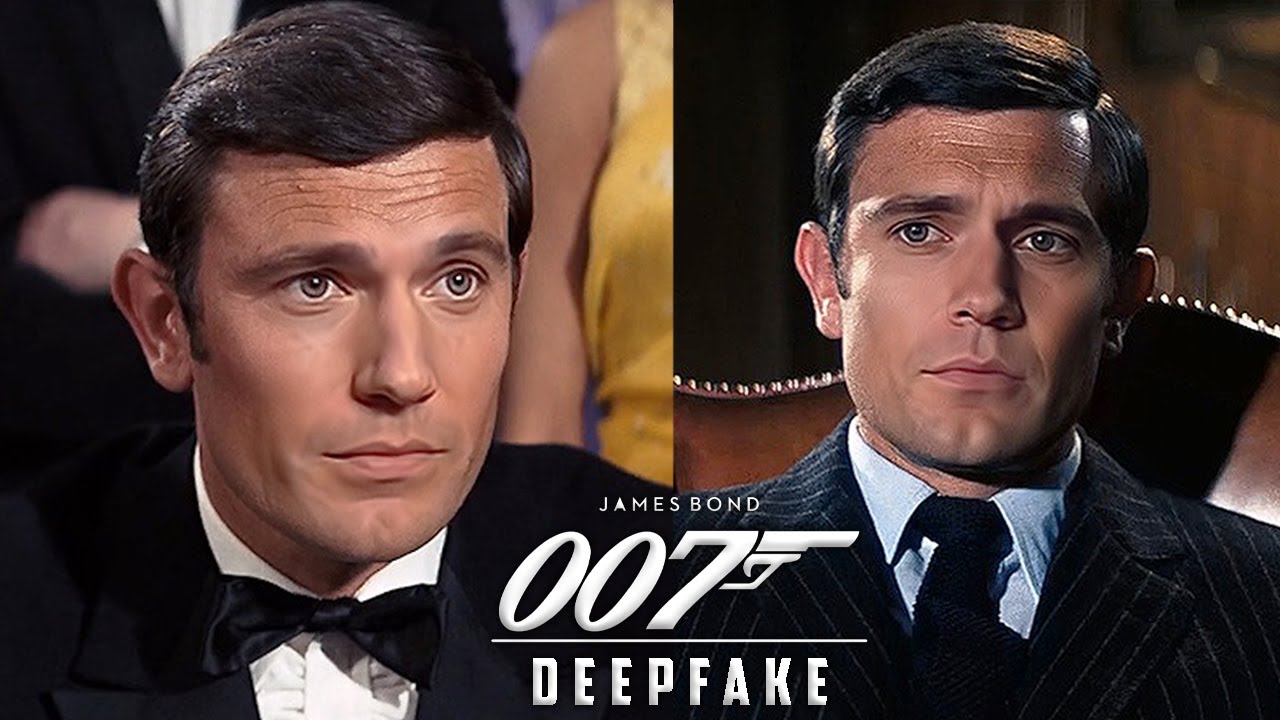The image showcases a side-by-side comparison labeled "James Bond 007 Deep Fake," suggesting a digitally altered or face-swapped portrayal. Both panels feature what seems to be the same man, indicating a deepfake technology application. On the left, the man is dressed in a classic black tuxedo with a white undershirt and a bow tie, his hair neatly combed back. Behind him, figures in formal attire, including a person in a yellow dress and another in a suit, populate the scene, hinting at a social or high-profile event. On the right, the same man, or a remarkably similar one, wears a striped suit paired with a blue shirt and a necktie. His hair is stylishly parted and combed to the left. In contrast to the left panel, the background here is nondescript, with no people visible, focusing entirely on his visage. This detailed comparison highlights the nuanced differences in attire, hairstyle, and background, underscoring the digital manipulation implied by the "Deep Fake" label.